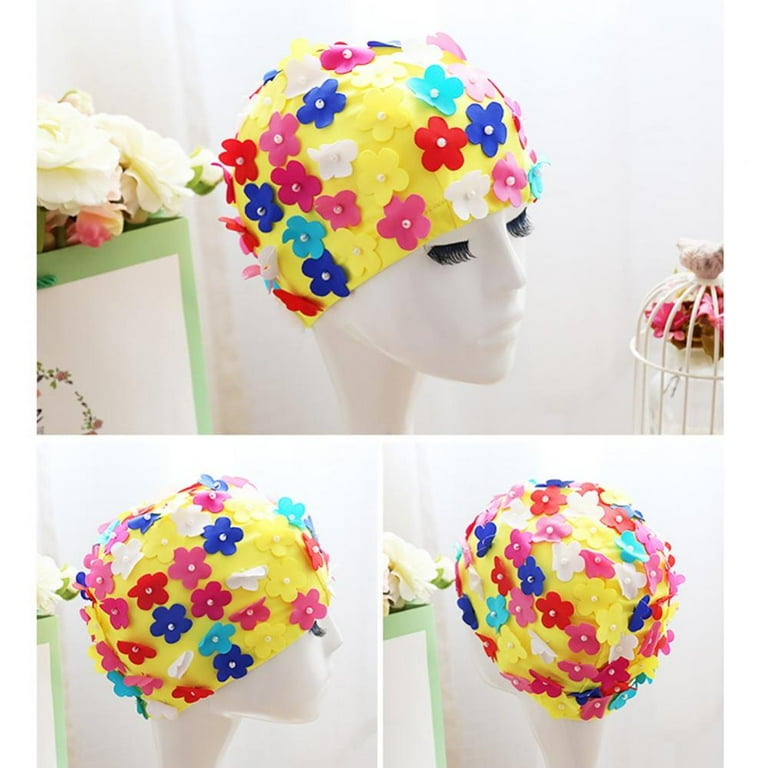The image features three views of a white mannequin head with black, thick eyelashes, displayed against a white background. The top half of the image showcases a larger, horizontal picture of the mannequin from the front, while the bottom half is divided into two square pictures showing different angles: a side view on the left and a back view on the right. The mannequin is adorned with a vibrant yellow shower cap, embellished with an assortment of colorful, plastic flowers, including pink, light blue, dark blue, yellow, and white flowers, which appear to be securely fastened onto the cap rather than painted on. Additionally, there are decorative items in the background, including a birdcage with flowers on the bottom right and a few flower arrangements on the back left.